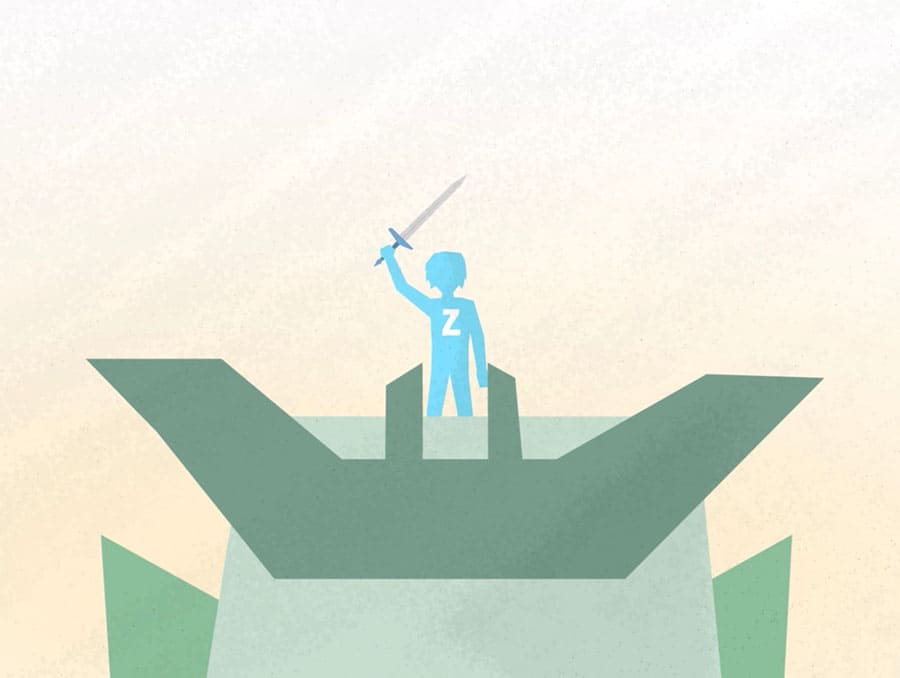This digital illustration features a simplistic, almost silhouette-like figure of a young male, centrally positioned, holding a grayish lilac sword aloft in a power pose. The figure is depicted in varying shades of light blue, adorned with a prominent white "Z" on the chest, though facial and hair details are minimally rendered. The background displays a blend of pink, white, beige, and gray hues, giving a sense of abstract or atmospheric backdrop. The figure stands on a large, green-and-beige platform, which may suggest a box, tank, or another elevated structure, with a darker-colored ledge in front of it. Flanking the scene on both sides are panels of greenish-gray, adding to the stylized, almost game-like aesthetic of the piece.